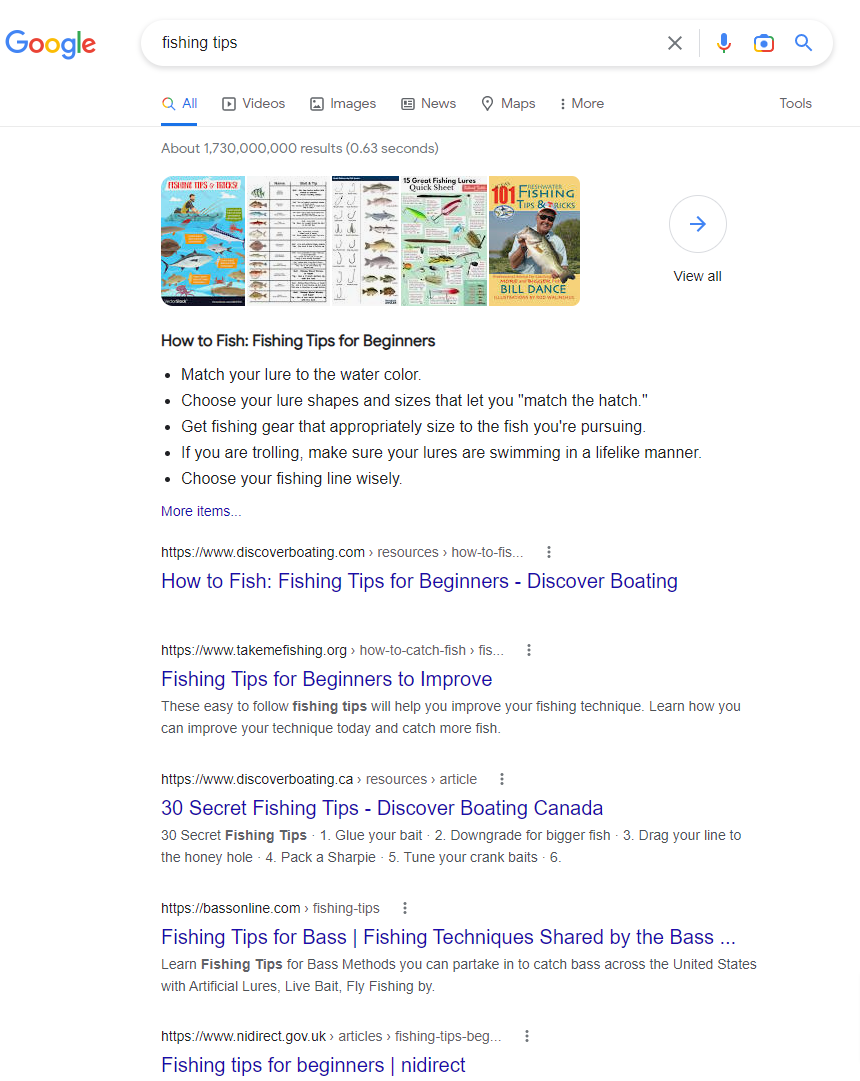Screenshot of a Google Search for Fishing Tips

This image is a screenshot displaying a Google search query for "fishing tips." At the top of the image, the search bar prominently shows the text "fishing tips," accompanied by the Google logo to its left. Directly beneath the search bar, there are several navigational tabs for categorizing the results: "All," "Videos," "Images," "News," "Maps," "More," and "Tools."

Immediately below these tabs, the search results indicate that there are approximately 1.7 billion results available, generated in just 0.63 seconds. Following this, five images are displayed, which appear to be diagrams, graphs, or guides related to fishing tips.

Continuing down the page, the AI-generated text box titled "How to Fish: Fishing Tips for Beginners" offers various tips for novice anglers. The tips include:
- Matching your lure to the watercolor.
- Choosing lure shapes that match the hatch.
- Selecting fishing gear appropriate for the size of the fish you're pursuing.
- Ensuring lures swim in a lifelike manner if you're trolling.
- Choosing your fishing line wisely.

Below the AI-generated tips, five specific website results are listed:
1. "How to Fish: Fishing Tips for Beginners" from Discover Boating.
2. "Fishing Tips for Beginners to Improve" (the source website is not specified).
3. "30 Secret Fishing Tips" from Discover Boating Canada.
4. "Fishing Tips for Bass: Fishing Techniques Shared by the Bass..." (the source website is truncated).
5. "Fishing Tips for Beginners" from an unspecified website, possibly directed to a Canadian context based on prior results.

Overall, this search seems to cater particularly well to individuals who are new to fishing and are looking for introductory advice, with a notable emphasis on Canadian resources and locations for fishing tips.